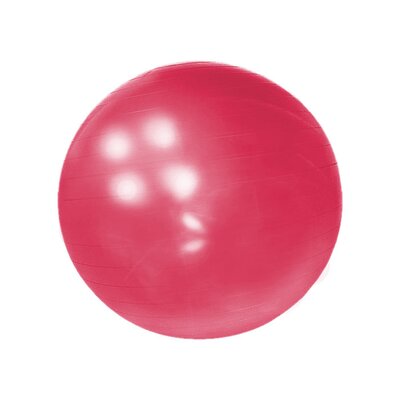The image features a light red, possibly dark pink, round exercise ball set against a plain white or black-and-white background. The ball displays faint horizontal lines scattered across its surface, providing structure and texture typical of an exercise ball. The lighting creates a reflection on the upper left side of the ball, marked by four prominent white circles and two smaller dots beneath them. These reflections highlight the smooth, inflated surface of the ball, which appears darker at the top and lighter at the bottom, with some white smudges or residue visible toward the base. The ball is not resting on any surface, giving it a stateless appearance.